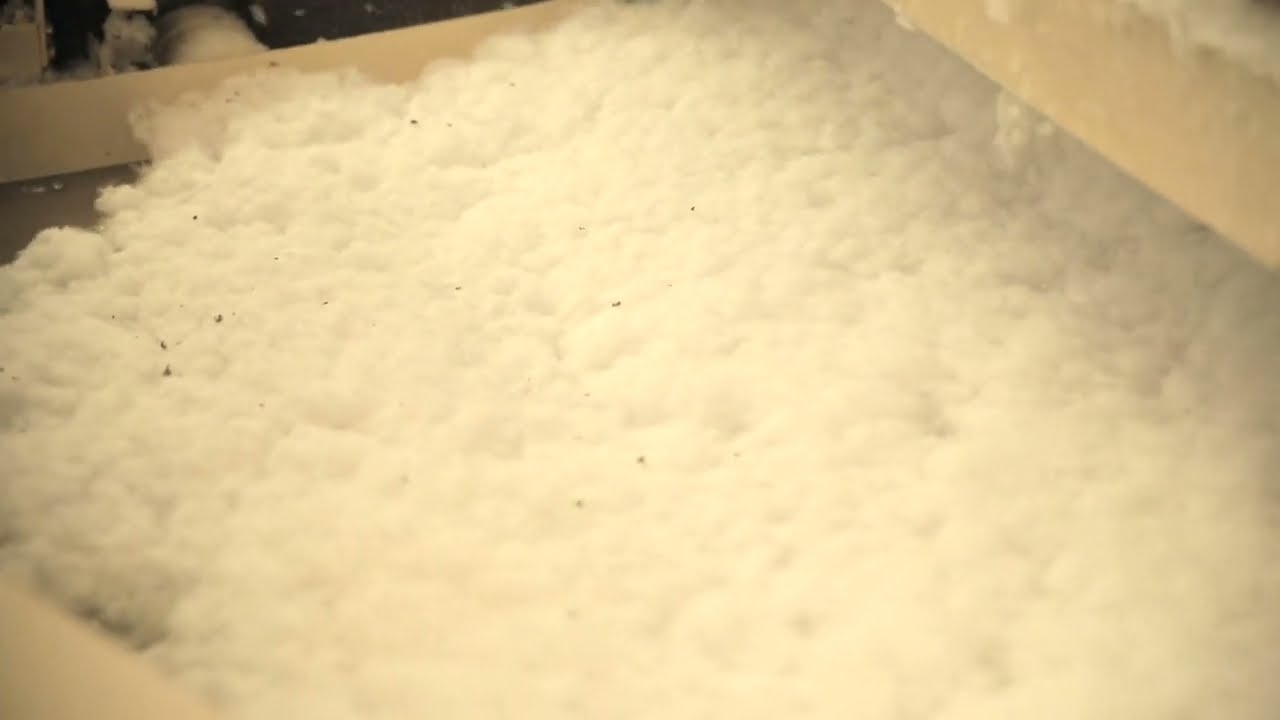The image depicts a predominantly off-white, nearly all-white scene that appears to be a close-up of a soft, fluffy material resembling a bed of cotton balls or possibly cushy foam. The texture looks uneven and non-smooth, similar to cotton batting. The cotton-like material is concentrated more towards the lower right and extends up towards the left, suggesting the camera's position is slightly off-center and to the right. In the top left corner, there seems to be part of a frame or the edge of a container, perhaps a flap folding inward, hinting that the material is within a kind of box or holder. This container is tan in color and includes some dirt specks, which might be on the lens. The top right corner shows some cotton possibly beginning to spill over or fall into another section. The scene is devoid of people or animals and the overall impression is one of a soft, cushioned expanse, evocative of either cotton balls, creamy foam, or even something like popped popcorn or rice.